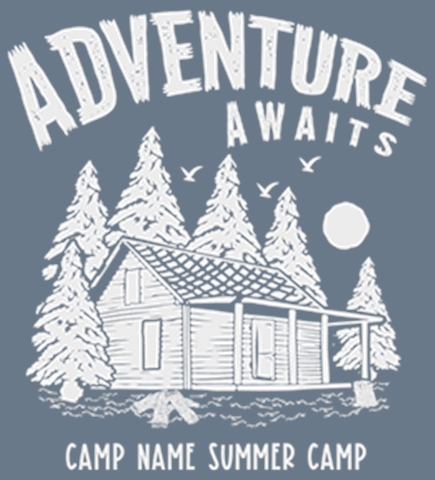The image is a vertically aligned rectangular poster with a solid dark gray background. At the top, large, all-caps white letters spell out "ADVENTURE AWAITS," with "AWAITS" in a slightly smaller font. Beneath this, a white illustration depicts a cabin with a covered porch, surrounded by pine trees. To the left and the right of the cabin are individual pine trees, with four additional trees situated behind it. A full moon appears above the right-side tree. Three birds, depicted as small V-shaped figures with horizontal lines at the bottom of each V, fly across the scene. Near the lower section of the image, logs arranged in a campfire setting are visible to the left of the cabin. Centered at the bottom of the poster, the text "CAMP NAME SUMMER CAMP" appears in all-caps white letters.